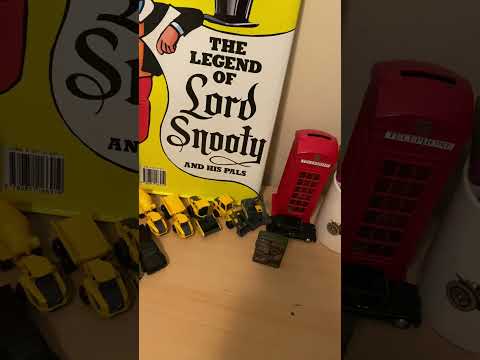This image depicts a light brown desk adorned with various items. Central to the scene is a white jar filled with multicolored magic markers, displaying an old automobile design. Positioned beside the jar is a miniature red British telephone box that appears to function as a coin bank due to the slot on its top. Also on the desk are small toy construction vehicles or Hot Wheels cars. Leaning against the beige wall at the rear, a book with a white and yellow cover prominently features the black-lettered title, "The Legend of Lord Snooty and His Pals." The background of the image is white, and the edges are bordered with enlarged, faded repetitions of elements from the central scene, adding a cohesive framing effect to the overall composition.